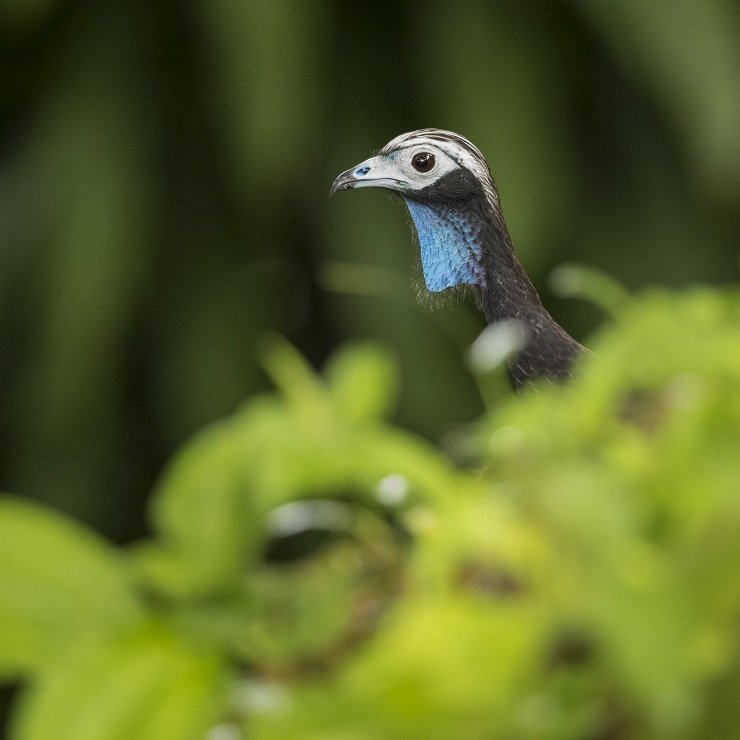This image captures the head and neck of a distinctive bird emerging from dense, blurred green shrubbery. The bird, positioned at the center of the photograph, is gazing towards the left. Its sleek neck is cloaked in dark gray, almost black feathers. The head is predominantly white with black-tinged accents, particularly around the cheeks and the tip of its white beak. Surrounding the bird's brown eye is a narrow ring of white, adding to its striking appearance. Notably, the area beneath the beak extending to the mid-neck features a unique blue patch, comprised of delicate, almost hair-like feathers, which appear as a blue-colored throat or gullet. The overall background is softly out of focus, drawing attention to the bird's distinct and vivid details.